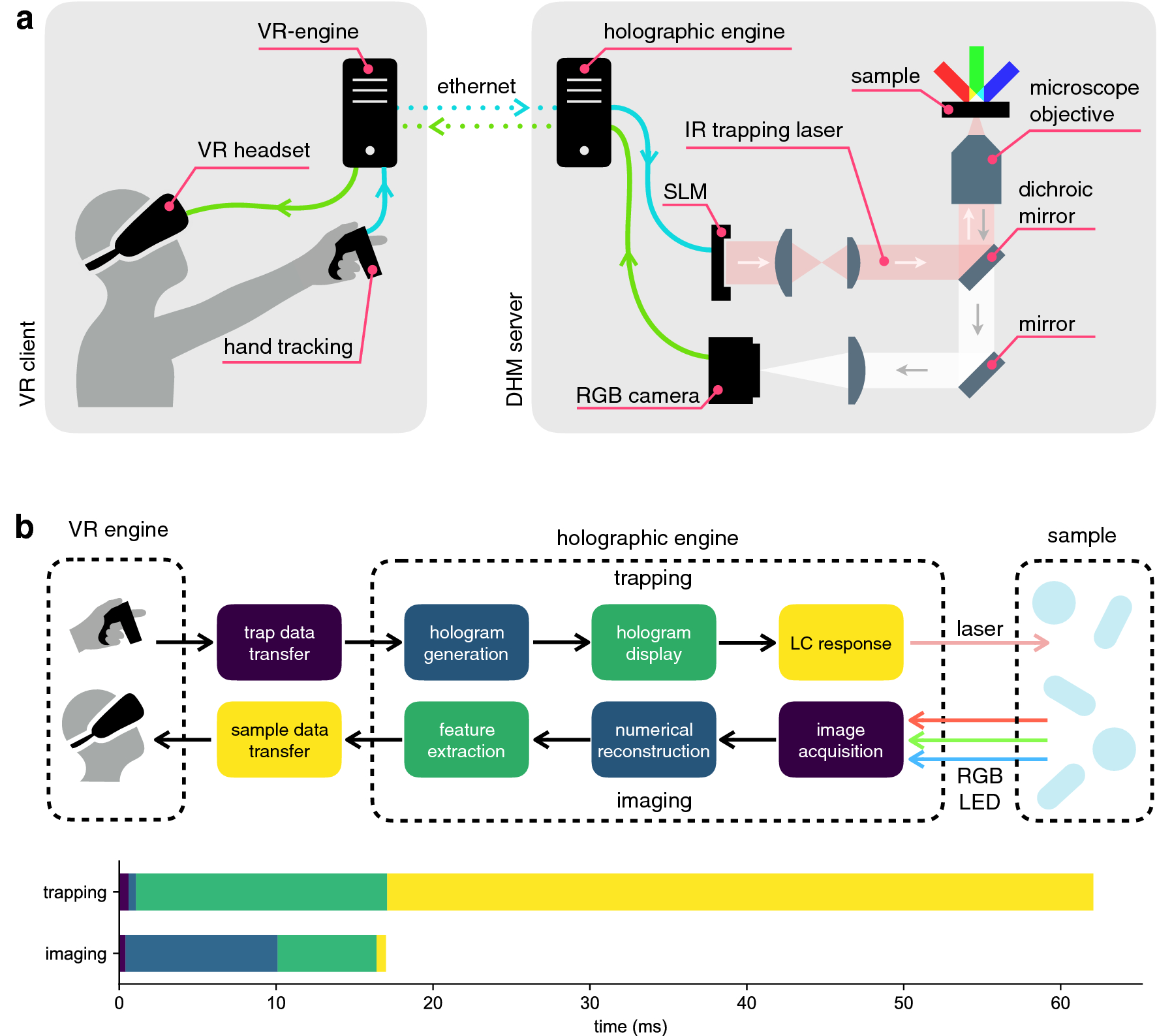The illustrated diagram is divided into two main sections labeled 'A' and 'B', each depicting different aspects of a VR system setup and operation. 

Section 'A', in the upper half, features a smaller box in the upper left corner with a lowercase 'a'. It contains a grey-shaded rectangular shape with rounded edges, displaying an outline of a person wearing a VR headset. There are prominent labels with red or pink lines pointing to specific parts: the VR headset on the person's head labeled "VR Headset," a remote in hand indicated as "Hand Tracking," and what appears to be a smartphone labeled "VR Engine." The box is connected to a larger grey-shaded rectangular box labeled "DHM Server" in the upper right corner by a two-way arrow composed of blue and green dotted lines, indicating an Ethernet connection. This larger box is detailed with several dark pink lines and terms like "Holographic Engine" (resembling another phone), "IR Trapping Laser" (represented by a beam), and additional components such as a mirror and an RGB camera.

Section 'B', in the lower half, starts with another lowercase 'b' on the left. It includes a vertical rectangular outline labeled "VR Engine," showing a hand holding the remote and a head with the VR headset. This is connected by two-way arrows leading to another rectangular section named "Holographic Engine," which includes multiple elements labeled "Hologram Generation," "Hologram Display," "LC Response," "Feature Extraction," "Numerical Reconstruction," and "Image Acquisition." Another series of two-way arrows extends from this to the rightmost rectangle labeled "Sample," topped with another "sample" title. Below, a sideways bar graph spans the entire section, with the x-axis ranging from 0 to 60 milliseconds. The graph has two bars: the top bar is color-coded green and yellow labeled "Trapping," and the bottom bar is blue, green, and a little yellow labeled "Imaging."

Overall, the diagram offers a comprehensive guide on setting up and understanding the connections between VR headsets, VR engines, hand tracking, and holographic engine operation, detailed with various components and data transfer pathways.